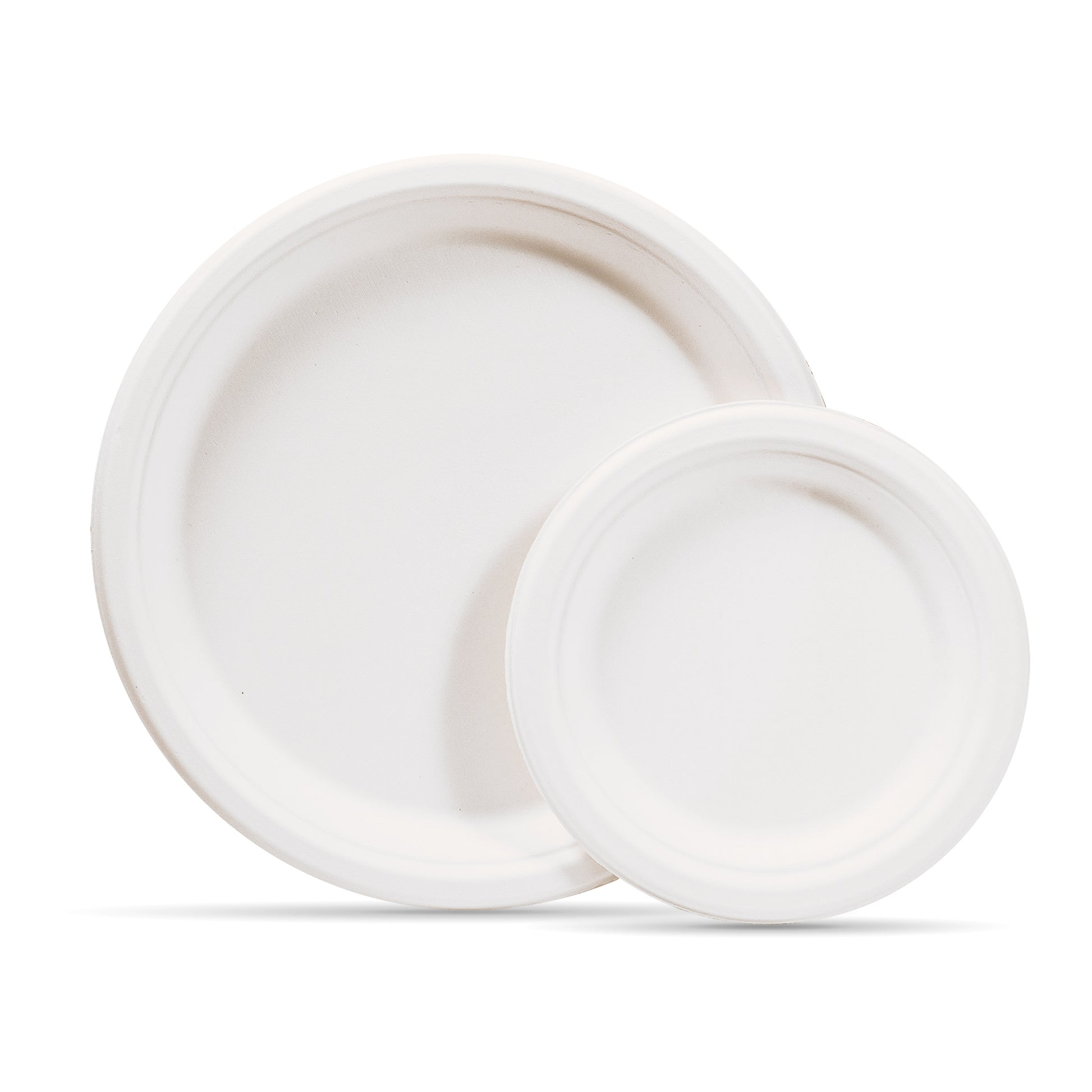The image features two white plates standing vertically against an all-white background, casting subtle shadows at their base. The larger plate, with a subtle lined border, is positioned centrally and slightly towards the back. In front of it, partially covering the larger plate, is a smaller, cake-sized plate located towards the right. The plates, which resemble paper or cardboard due to their texture and design, appear to be illuminated by natural light, making the setting bright and the details of the plates clear. The image is free of any text or additional objects, emphasizing the simplicity and clarity of the display.